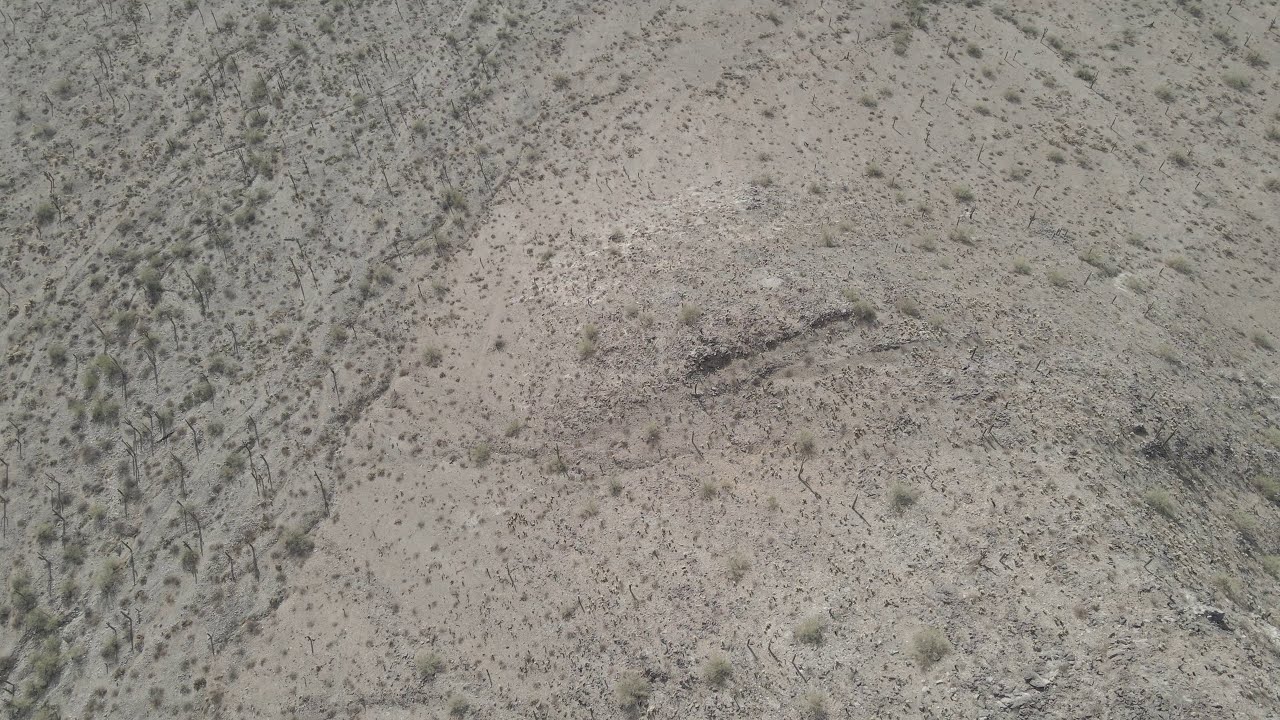This horizontally rectangular, high-definition photograph captures an aerial view, taken from a significant altitude, possibly from an airplane or high in the Earth's atmosphere. The landscape below resembles a desert or sandy area, predominantly brown with patches of green vegetation scattered throughout. The vegetation includes trees, shrubs, and weeds, which appear as tiny specks from this height. Notably, in the center of the image, there is what seems to be a large, non-human footprint imprinted in the sand. This footprint adds a focal point to the otherwise barren terrain. The left side of the photograph shows a denser cluster of greenery, contrasting with the more sparsely vegetated, sand-dominated center. The right side also features scattered green patches. There are no visible buildings or people in the image, and the scene is taken in daylight, giving it a realistic appearance, though it's unclear if this is a photograph or a highly detailed painting due to its intricate details.